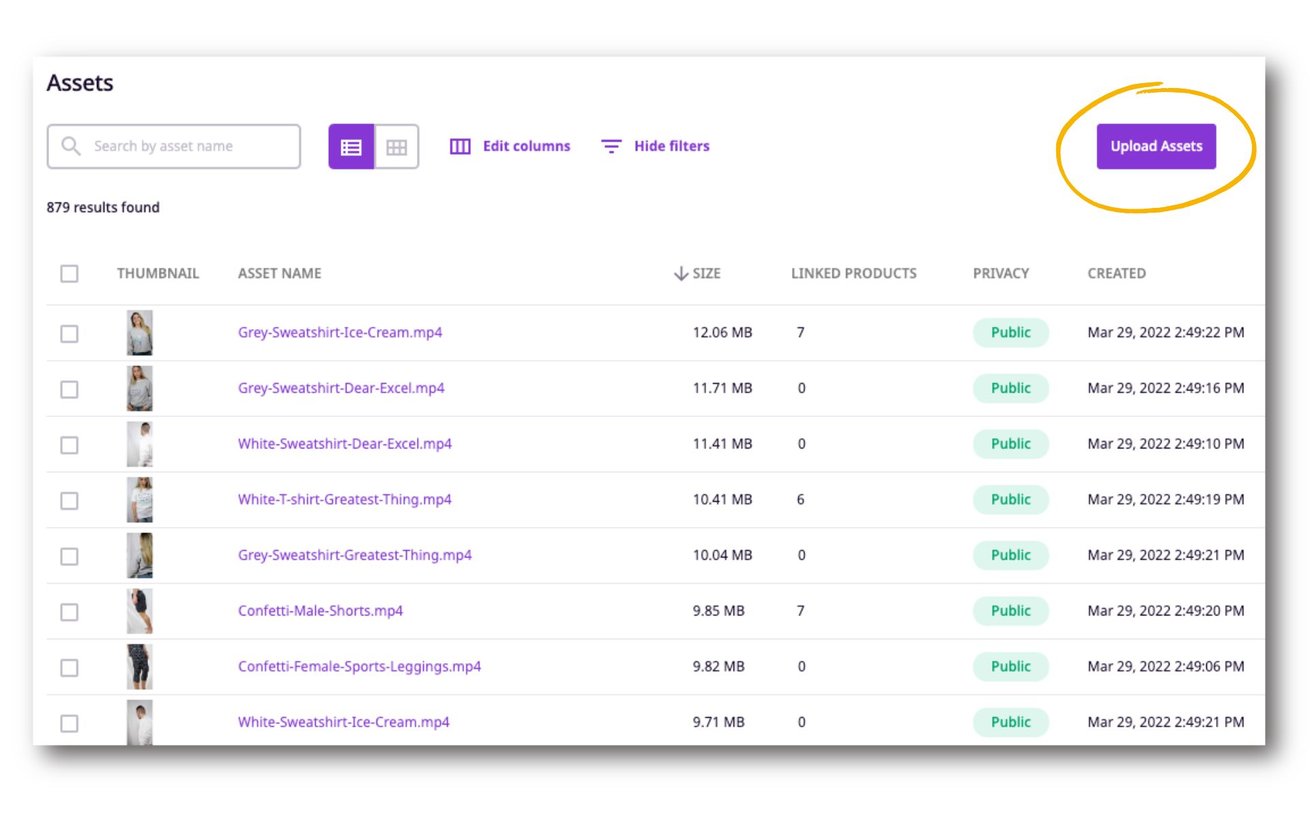The image depicts a white webpage with a minimalist design and purple text. In the top left corner, there is the word "Assets" displayed prominently, directly below which lies a search box for easy navigation. On the top right corner, there is a purple button labeled "Upload Assets," encircled with a hand-drawn yellow ring to highlight its importance.

The main section of the page consists of a table with multiple columns labeled: "Thumbnail," "Asset Name," "Size," "Linked Products," "Privacy," and "Created." The "Thumbnail" column displays images of women modeling various white shirts, pants, and other apparel. The "Asset Name" column lists names such as "Gray Sweatshirt" and "Ice Cream," indicating the titles of different assets, all of which are MP4 files. 

The "Size" column shows a range of file sizes from 9 MB to 12 MB. The "Linked Products" column includes numerical values, presumably indicating how many products are associated with each asset. The "Privacy" column lists all items as "Public." Lastly, the "Created" column records the creation dates of these assets.

Overall, the webpage is an organized and user-friendly interface for managing multimedia assets, complete with clear sections and functional search and upload options.